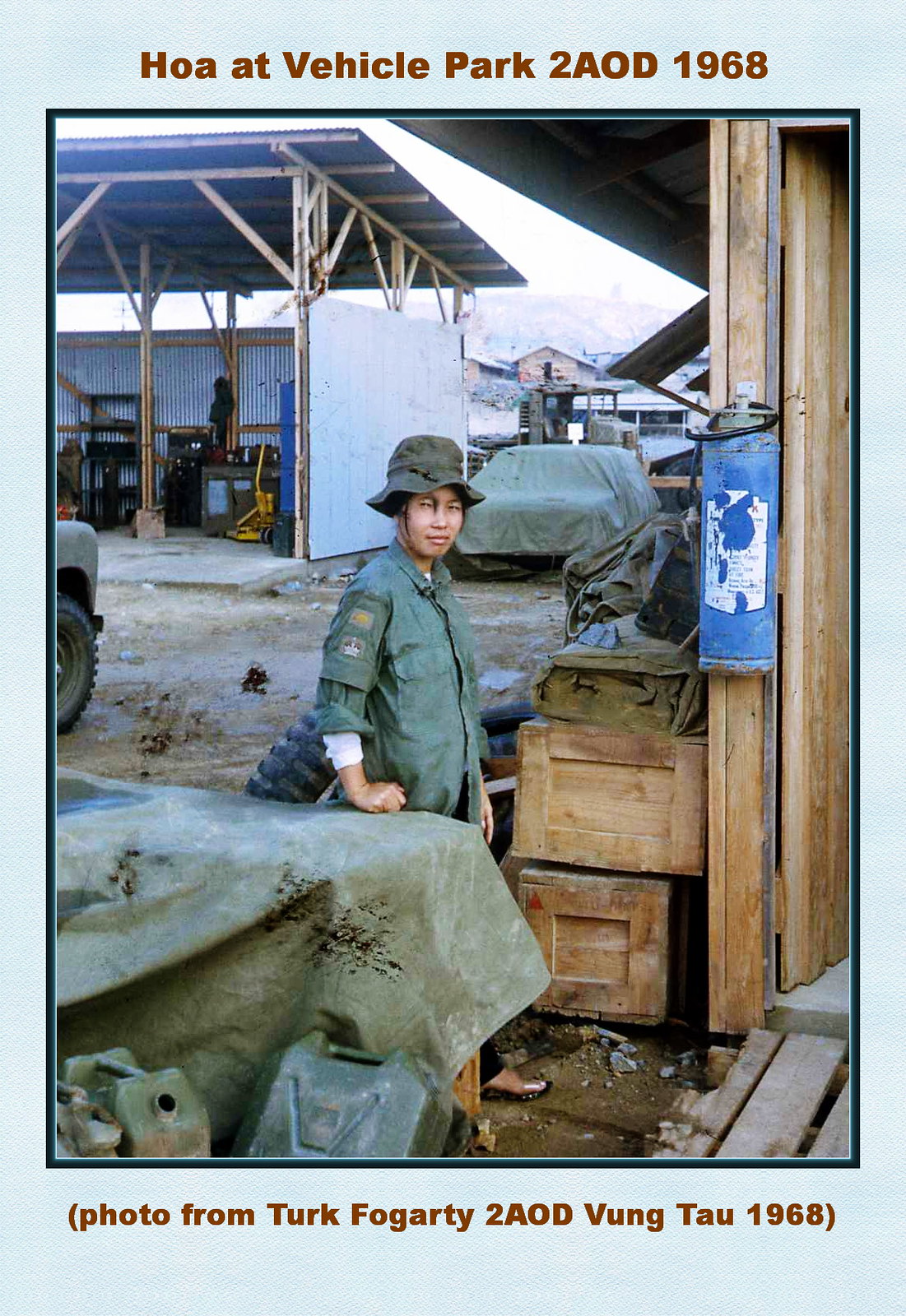This photograph, framed with a green border against a light blue background, depicts an Asian-looking individual in a military setting in Vung Tau, 1968, as noted by the text reading “HOA at Vehicle Park 2AOD 1968” at the top and “Photo from Turk Fogarty to AOD Vung Tau 1968” at the bottom. The person, dressed in olive-green military fatigues and a slightly floppy brimmed hat, stands in a garage-like area amidst a collection of military equipment. Their body faces right, but their gaze is directed towards the camera. Surrounding them are crates, tarps, and scattered gasoline cans, with a green-tarp-covered vehicle nearby. The scene also includes a blue fire extinguisher to the far right and a metal building with a wooden frame, indicating a makeshift yet functional setup. This detailed image captures a moment of daily life on a military base, offering a glimpse into the environment and conditions of the time.